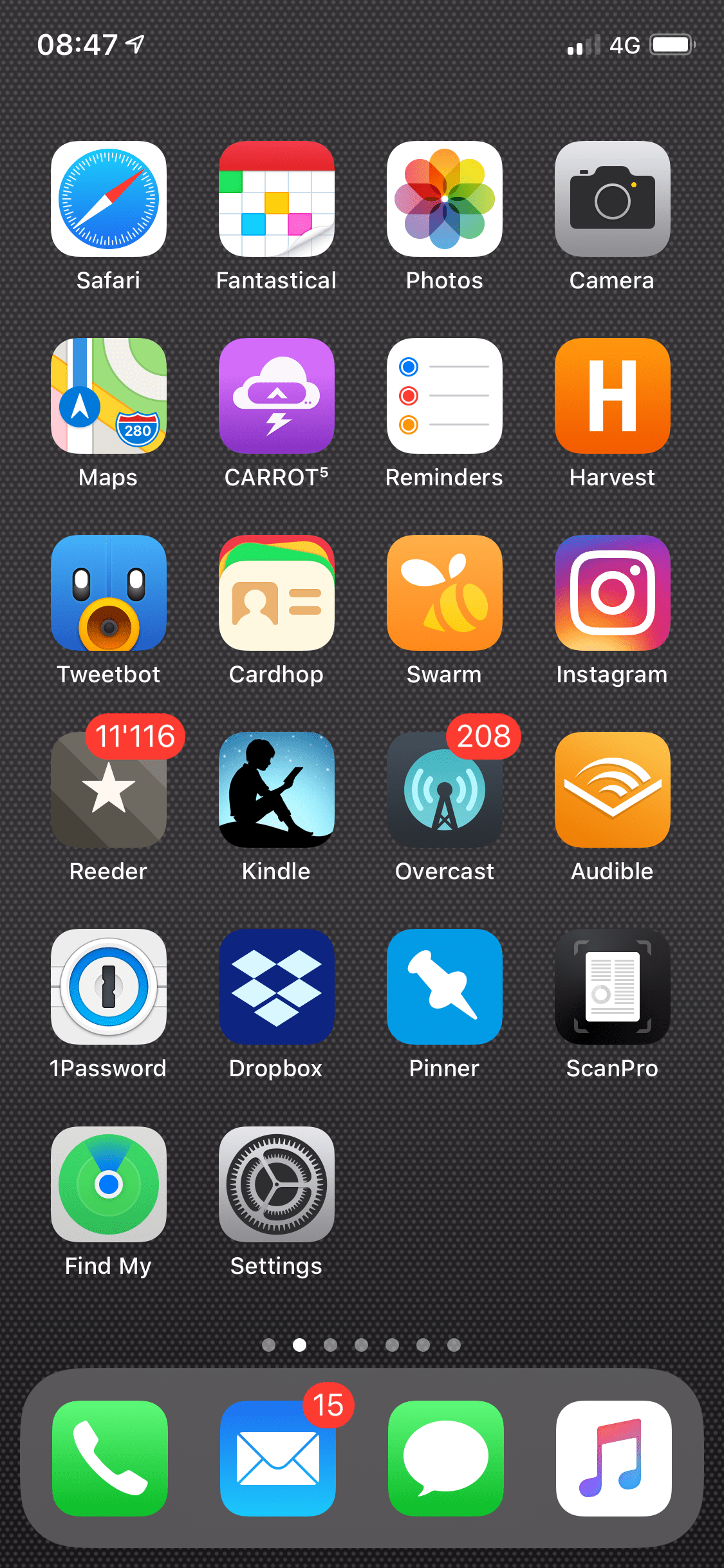The image is a screenshot of a cell phone's home screen set against a black backdrop. In the upper left corner, white text displays the time as 8:47. The upper right corner shows two out of four signal bars, indicates a 4G connection, and a fully charged battery icon. The home screen showcases several app icons arranged in a grid format. The first row features Safari, Fantastical, Photos, and Camera. The second row includes Maps, Carrot, Reminders, and Harvest. The third row displays Tweetbot, Cardhop, Swarm, and Instagram. The fourth row contains Reader, Kindle, Overcast, and Audible. Finally, the fifth row has 1Password, Dropbox, Pinner, and ScanPro, followed by the icons for Find My and Settings.